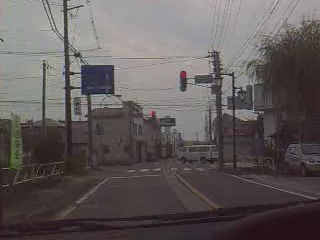This photo, taken through the windshield of a car with a black or dark gray dashboard and visible windshield wipers, depicts a European urban street scene. The vehicle appears to be driving on the left side of the road, pointing to a likely European location. On the left side of the street, there is a guardrail alongside a gray concrete median, followed by a yellow divider and white edge lines marking the boundaries of the road. To the right, a small, older car is parked in front of a building surrounded by overgrown grass and trees. In the distance, a blue freeway sign is visible, mounted on a pole. Scattered electrical line poles and a red traffic light, mounted on an upside-down L-shaped pole, add to the urban landscape. Ahead, a white truck is making a right turn from a side street. The sky overhead is gray and cloudy, indicating overcast weather.